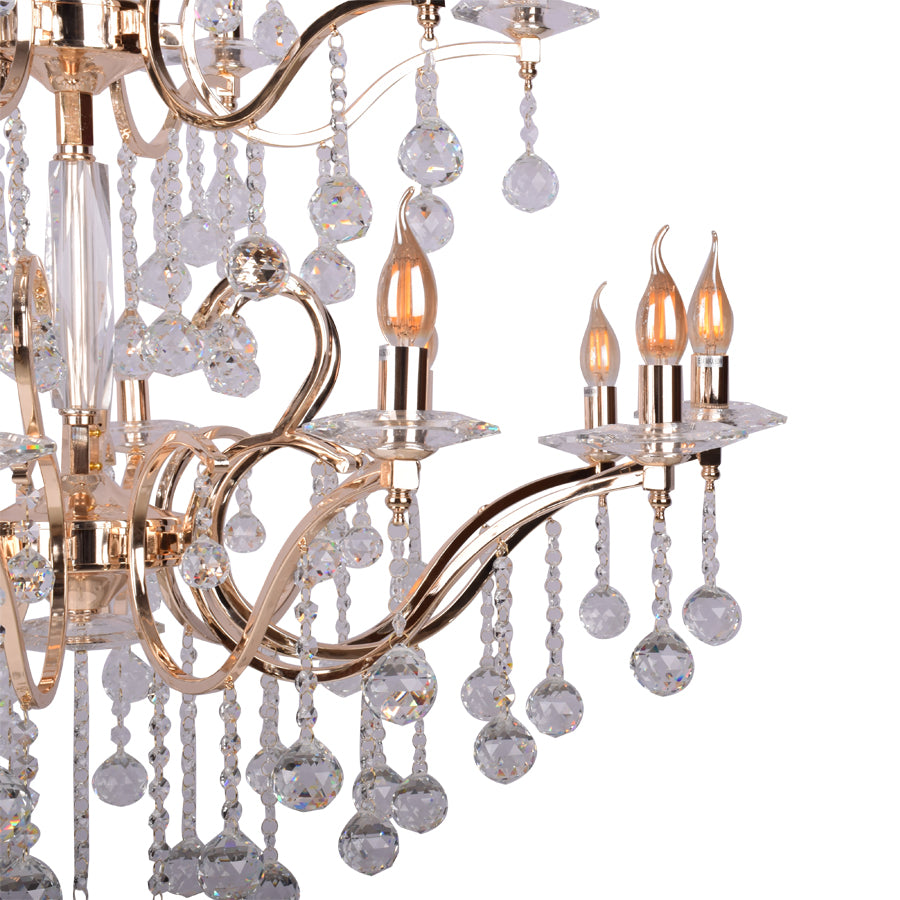The photograph showcases a portion of an ornate white and pink gold brass chandelier, commonly found in affluent settings such as grand dining rooms or living rooms. The chandelier's design features flowing, soft curves with intricate details. Central to the image, we see a large, rectangular centerpiece made of crystal that connects the various components of the chandelier. Attached to it are numerous small flame-shaped LED bulbs that emit a yellowy-orange glow, mimicking the appearance of real flames.

The chandelier is adorned with multiple layers of dangling crystals, each set suspended from delicate chains. The crystals vary in size, with sequences ranging from two to six smaller crystals culminating in a larger crystal at the end of each strand. Adding to the opulence, these crystals are clear, off-white in color, and their shimmering quality is highlighted by the chandelier's pink gold and brass framework.

Notably, there are at least four flame-tipped bulbs, with one central bulb and three positioned to the right. Below these bulbs, more crystal ornaments dangle, enhancing the chandelier's luxurious appearance. The chandelier stands out vividly against a white background, emphasizing its intricate details and elegant craftsmanship.